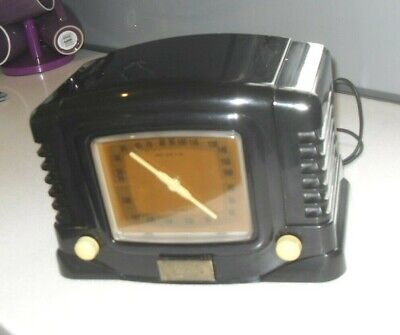This image features a close-up of a vintage Bakelite device, reminiscent of mid-20th-century design, possibly from the 40s, 50s, or 60s. The item is black and shaped like a small toaster, with a rounded top and a boxy structure. On either side of the device, there are white or off-white knobs. The front hosts a circular dial, which resembles a clock face with two hands – one at the 9 o'clock position and the other at 4 o'clock. The face of the dial has a weathered appearance, colored in a dark mustard yellow or burnt orange hue. Below the dial, there is a silver square plate that might be a signature plate, a decal, or simply a decorative element. The device seems aged or intentionally crafted to look vintage and might serve as a clock, a radio, or another type of measuring instrument. It is placed on a white countertop, with purple or cranberry-colored mugs visible in the background, and a bluish beige gray wall. This context implies a kitchen or household setting.